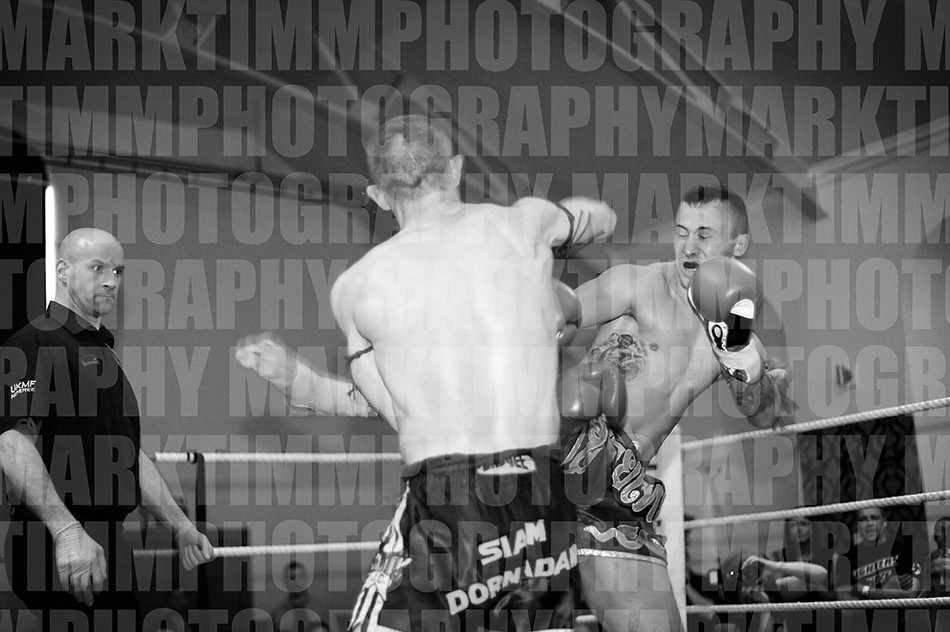In this black and white image of a kickboxing match, two Caucasian kickboxers are the focal point, captured mid-action in a ring. The boxer closest to the camera, wearing black shorts with white stripes and barely visible white lettering that reads "SLAM, DORN DARE," has his back turned. He has short brown hair, and black straps around his arms just below the shoulder. His opponent is delivering a roundhouse kick to his upper arm area. This kicking boxer also wears black shorts with gray lettering, has a tattoo on his left chest under the shoulder, and keeps one boxing-glove-clad hand raised near his mouth for defense.

The scene is set within the delineating ropes of the ring, with a bald referee in a black shirt to the far left, his hands positioned low by his hips. The referee's shirt bears the white text "UCMF." In the background, spectators watch the intense match unfold. Overlaying the entire image is a watermark that reads "Mark Tim Photography," repeated from top to bottom, ensuring the attribution is unmistakable.